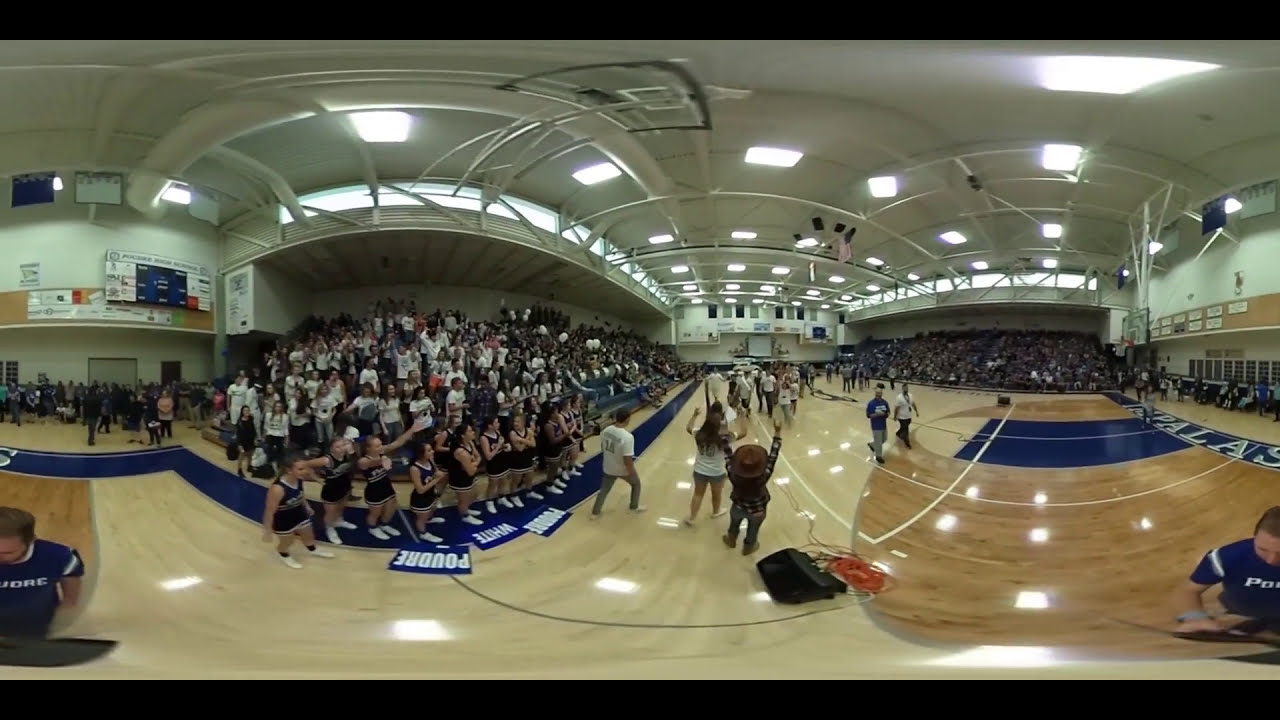The image captures a high school pep rally or sports event held in a spacious gymnasium, viewed through a lens that creates a distinct fishbowl or circular distortion. The scene features a large crowd of people filling the bleachers, predominantly visible on the left, likely composed of students. In the forefront, a group of cheerleaders dressed in blue uniforms stands near signs with the word "POUDRE" in large white letters, indicating the school's name. Central to the image, a person dressed as a cowboy raises their hands in mid-gesture. The photo has multiple visual centers due to the lens distortion, making it appear as if similar scenes are repeated on the left and right sides. The gym's ceiling is lined with numerous lights, and the floor consists of various shades of blue and brown, creating a dynamic backdrop for the event.